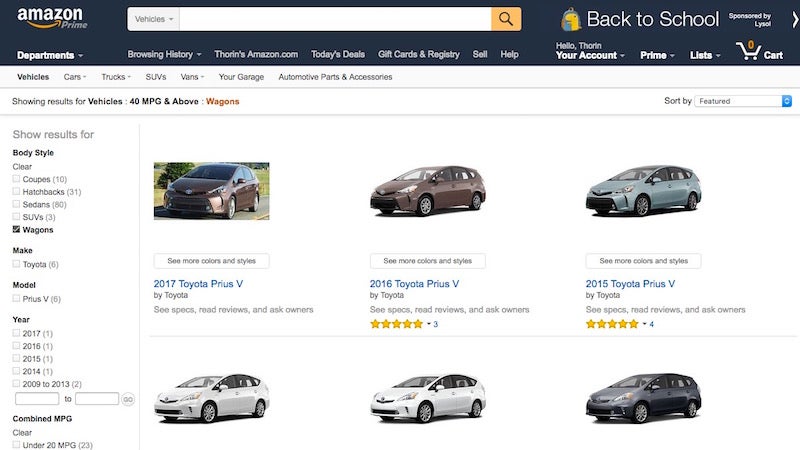Screenshot of an Amazon webpage showing an apparent search for vehicles. The top section of the screenshot features a black background with the Amazon logo and the orange smile arrow underneath it. To the right of the logo, "Prime" is displayed in gray font. Below this, there is a search bar where someone has entered "vehicles."

On the right side of the top section, there's a yellow backpack image with white text indicating "Back to School," alongside a note mentioning sponsorship by Lysol. Below this section, navigational links are visible, including "Departments," "Browsing History," "Amazon.com," "Today’s Deals," "Gift Cards," "Registry," "Sell," and "Help." 

A greeting "Hello, Thorn" appears, followed by options for "Account" and "Prime listings." The cart icon shows that it is empty. In the main content area, a white background with gray text lists categories such as "Vehicles," "Cars," "Trucks," "SUVs," "Vans," "Your Garage," and "Automotive Parts and Accessories."

Moving further down, there are filters for vehicle search criteria, including "Body Type" (Coupe, Hatchback, Sedans, SUVs, Wagons), "Make" (highlighting Toyota Prius), and "Year" options spanning from 2017 to 2009-2013. Additionally, a filter for combined MPG rating, displaying options under 20 MPG and above 25 MPG, is present.

Three vehicle listings are shown on the page, predominantly Toyota Priuses. The first listing features an image of the vehicle driving down a road, while the remaining two listings display vehicles on a white background.